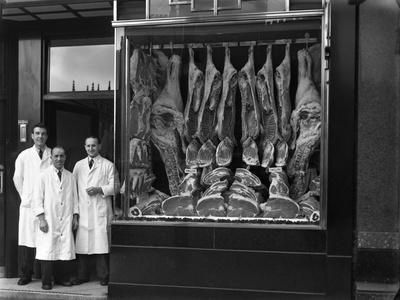This black-and-white photograph, possibly from the 1950s or earlier, captures a detailed scene of a butcher shop's front display. Central to the image are three men, all dressed in immaculate white coats, black trousers, and ties, standing in the shop's entryway. The man on the left is tall with dark hair, the middle man is shorter and balding, while the third, of medium height, also appears to be losing hair. They stand smiling at the camera, their formal attire of lab coats or smocks contrasting against the backdrop of the shop. 

To their right, a large refrigerated display window spans the front of the shop. Inside, various cuts of meat, likely pork, are meticulously arranged. Rows of large meat pieces hang from hooks on a rod, and additional cuts lie organized at the bottom of the display. Visible details include hooves, open areas of meat, name tags, price indicators, and identifier tags, all contributing to the meticulously presented assortment. The shop window, refrigerated to maintain the meat, allows a clear view of the substantial cuts suspended and displayed below.